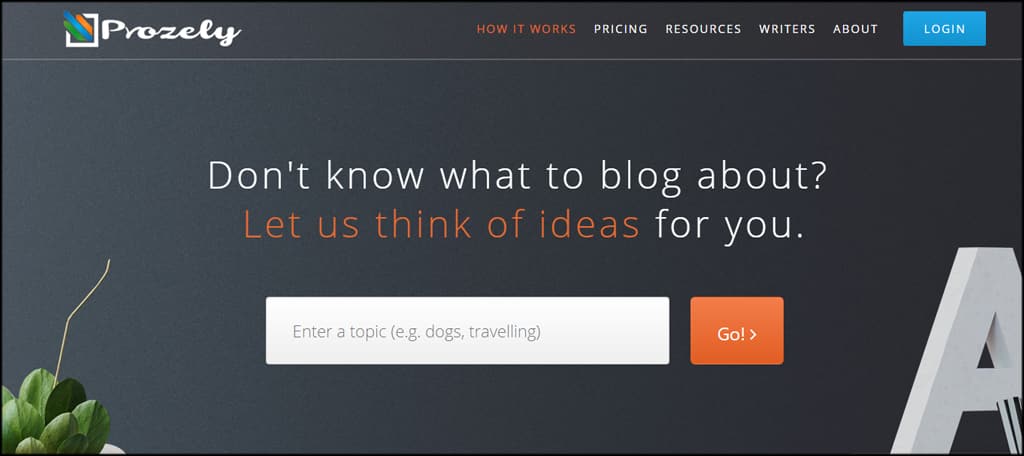The horizontal image features a predominantly gray background with minimal texture, providing a flat, one-dimensional appearance save for some light shadows and glares on the left side. In the upper left corner, a white box displays 'Prosely' in a white script font with green, blue, and orange lines emerging from it. To the right, an orange text reads "How it works," followed by white text options: "Pricing," "Resources," "Writers," and "About." A blue button labeled "Log in" in white font is also present.

The central section is divided by a thin white-gray line. The text within this section reads "Don't know what to blog about" in white, followed by "Let us think of ideas" in orange, and concluding with "for you" in white again. Beneath this, there's a white search box with placeholder text "Enter a topic, example: dogs traveling." Beside it is an orange button that says "Go."

In the bottom left corner, a green plant with a small stem is visible. The bottom right corner features a large, bubble-style letter "A" protruding slightly from the corner.